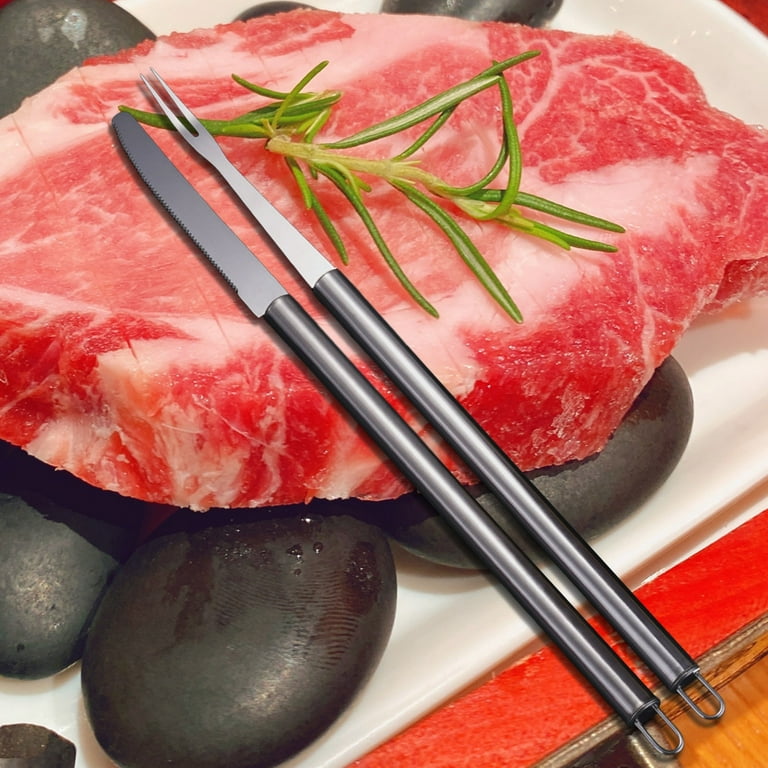The photograph is a vibrant, high-quality close-up of an uncooked, oval-shaped steak, rich in deep red hues with marbling of white fat. The steak is placed on a bed of black, pebble-like cooking stones, which rest on a white dish that extends slightly out of frame. A sprig of green herb, possibly parsley or cilantro, adorns the top of the steak. Diagonally across the steak, from the back left to the front right, are two slim, black metal utensils: a serrated knife with a rounded handle and a matching two-pronged fork. The scene is set against a red surface that peaks out from underneath the white dish. In the bottom right corner, there is a small piece of layered wood. The image beautifully captures the textural details and contrasting elements, emphasizing the rich colors and the assorted elements that make up this culinary presentation.